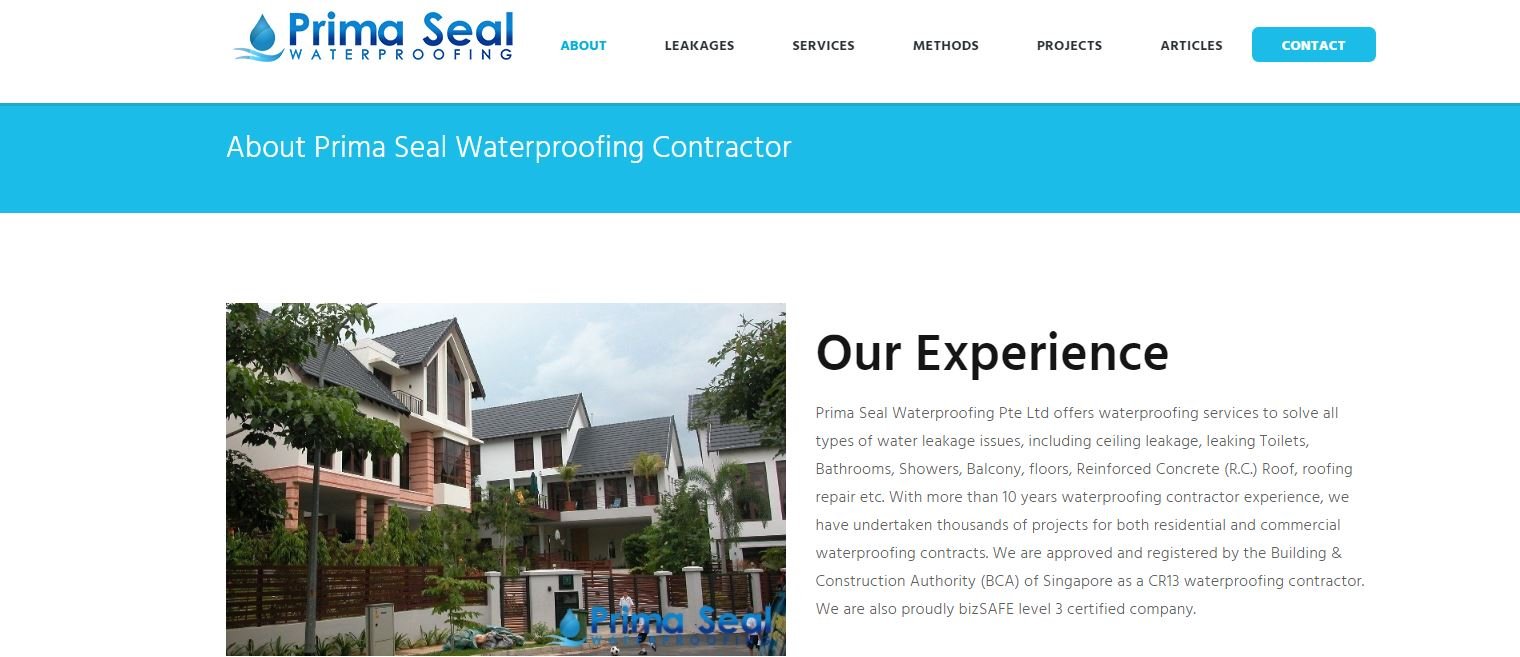A screenshot of a website titled "PrimaSeal Waterproofing" is displayed. At the top left, the PrimaSeal logo prominently features a water droplet above two simple wave-like lines, symbolizing water. The text "PrimaSeal" is larger and sports a gradient color scheme that transitions from a lighter blue at the top to a darker blue at the bottom, while "Waterproofing" is in smaller, solid black letters beneath it.

To the right of the logo, the website's menu is highlighted. The "About" section is marked in blue text, standing out against the other menu items—"Leakages," "Services," "Methods," and "Articles"—which are in black text. Further to the right, a blue button labeled "Contact" in white text completes the menu.

Below the menu, a large blue stripe runs horizontally across the screen with the white text "About PrimaSeal Waterproofing Contractor" prominently displayed. Directly beneath this stripe, a photograph showcases modern townhouses, with the PrimaSeal logo stamped in the bottom right-hand corner of the image.

To the right of the photograph, the section titled "Our Experience" includes a paragraph detailing their services, although the text is light and small, making it difficult to read clearly. The design of the website appears very generic with a simplistic layout and some arguably strange design choices, contributing to an overall plain and uninspiring aesthetic. The lower part of the screenshot remains blank, adding to the minimalistic yet bland feel of the site.